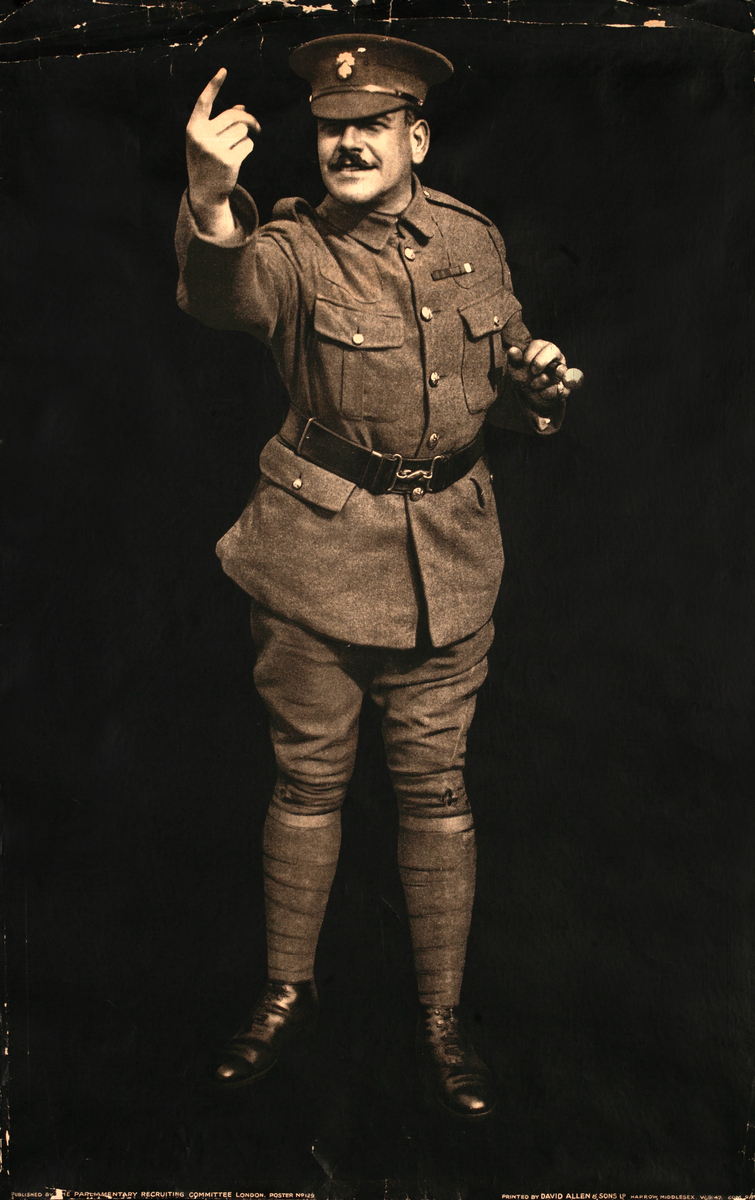In this black-and-white or sepia-toned photographic image, an older-looking poster of a soldier is seen affixed to a dark, nondescript backdrop, detailed with visible creases and lines from being folded and unfolded. The man, who bears a resemblance to Joseph Stalin, is depicted in a formal military attire, indicative of an older era. He wears a high-necked coat fastened with single buttons and cinched at the waist with a black belt. His ensemble includes matching pants and footwear, likely boots. The soldier dons a peaked military cap adorned with a small insignia on the front. Exhibiting a stern demeanor, he has a dark mustache and is looking slightly away from the camera, adding to his authoritative presence. His left hand is raised to chest level, with his middle and index fingers extended in a commanding gesture, while a baton is tucked under his left arm. The overall composition suggests an air of solemnity and order, underscored by the image's aged and weathered appearance.